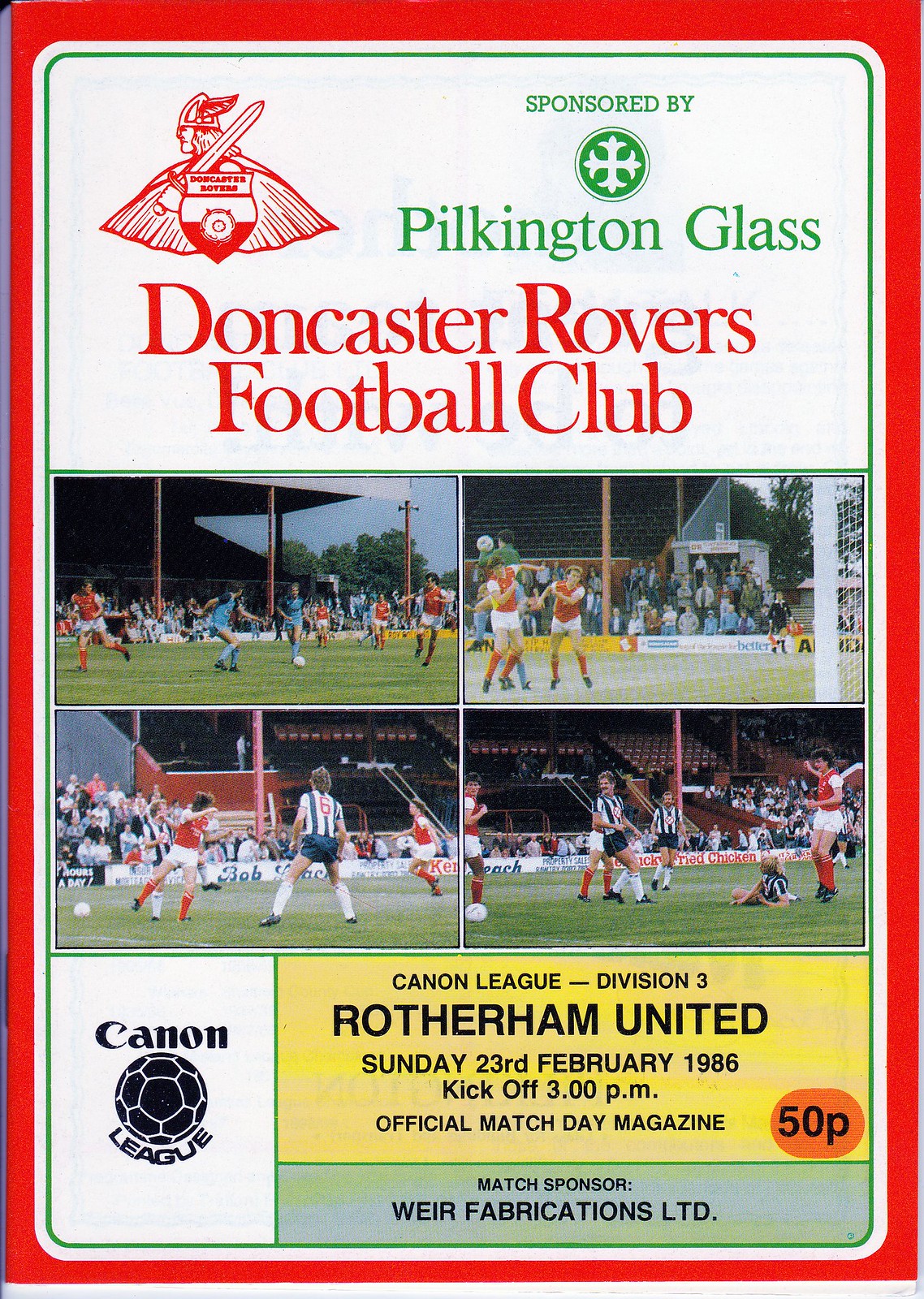This vintage football program, bordered in red with an additional inner green line, showcases a detailed layout against a white backdrop. In the upper left-hand corner, the Doncaster Rovers logo features a Spartan-like figure in a winged helmet, brandishing a sword and holding a shield, with a cape draped on his back. Adjacent to this, in green text, is "Sponsored by Pilkington Glass," accompanied by the green and white Pilkington Glass logo. Below, in prominent red letters, the title "Doncaster Rovers Football Club" is centered.

The central portion of the program is a collage of four photographs depicting soccer matches played under a clear blue sky. The images highlight players in different team kits: red jerseys with white shorts, blue jerseys with blue shorts, and white jerseys with blue stripes paired with blue shorts. The audience and stadium stands are visible in the background.

At the bottom left, a logo of the Canon League stands out with a black soccer ball separating the words "Canon" and "League." To the right, in a yellow rectangular box, details of the match are printed: "Canon League Division 3, Rotherham United, Sunday 23rd February 1986, kickoff 3 p.m. official match day magazine." An elongated orange oval displays the price "50p." Finally, along the bottom, a green strip announces the match sponsor, "Weir Fabrications Limited."